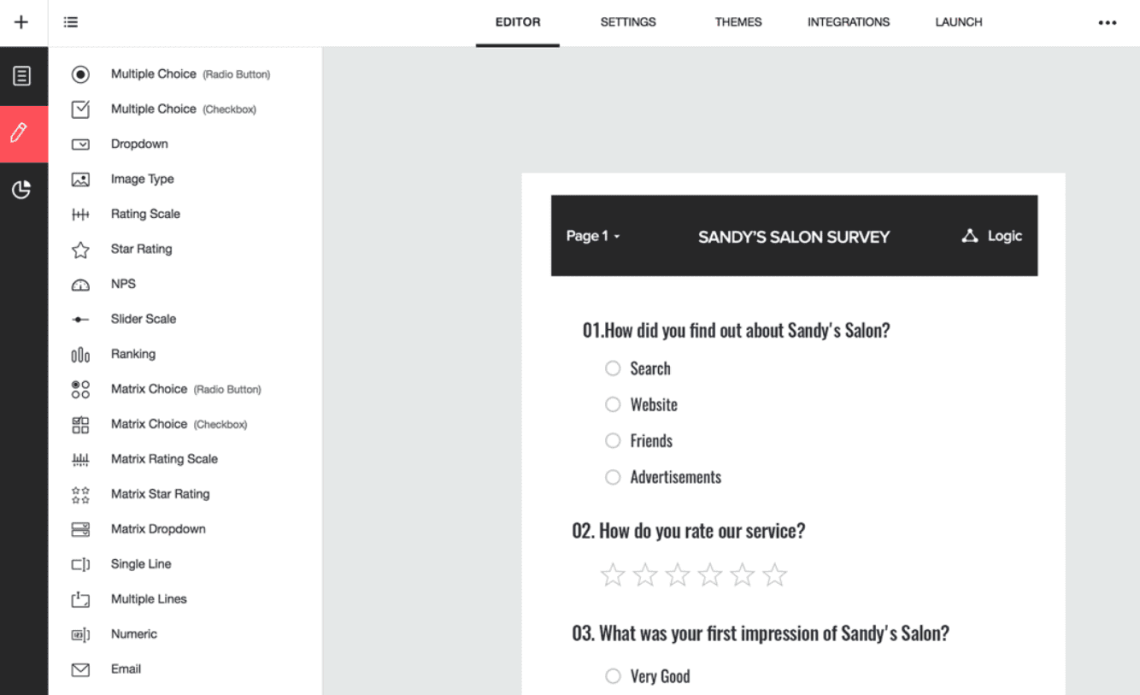The image depicts the interface of an online survey creation tool. At the top, a set of icons is visible, each representing different question types: a red pen icon, a circle, and black text options such as Multiple-Choice (Radio Button), Multiple-Choice (Checkbox), Drop-down, Image Type, Rating Scale (Star Rating), Net Promoter Score (NPS), Slider Scale, Ranking, Matrix Choice (Radio Button), Matrix Choice (Checkbox), Matrix (Rating Scale), Matrix (Star Rating), Matrix (Drop-down), Single Line, Multiple Lines, and Numeric Email.

Below the icons, the editor's toolbar displays options including Editor, Settings, Themes, Integrations, and more (indicated by an ellipsis).

Central to the image is a gray square section containing text on a white and black background. The text reads: "Page 1: Sandia Salon Survey," followed by logic statements and question IDs such as "0-1. How did you find out about Sandia Salon?" with checkboxes for response options 'Search,' 'Website,' 'Friends,' and 'Advertisements,' all currently unchecked.

Another question reads: "0-2. How do you rate our service?" with response options ranging from 1 to 6 stars.

The subsequent question, "0-3. What was your first impression of Sandia Salon?" includes a text box for open-ended responses.

Overall, the image showcases a detailed survey for Sandia Salon that is in the process of being designed.